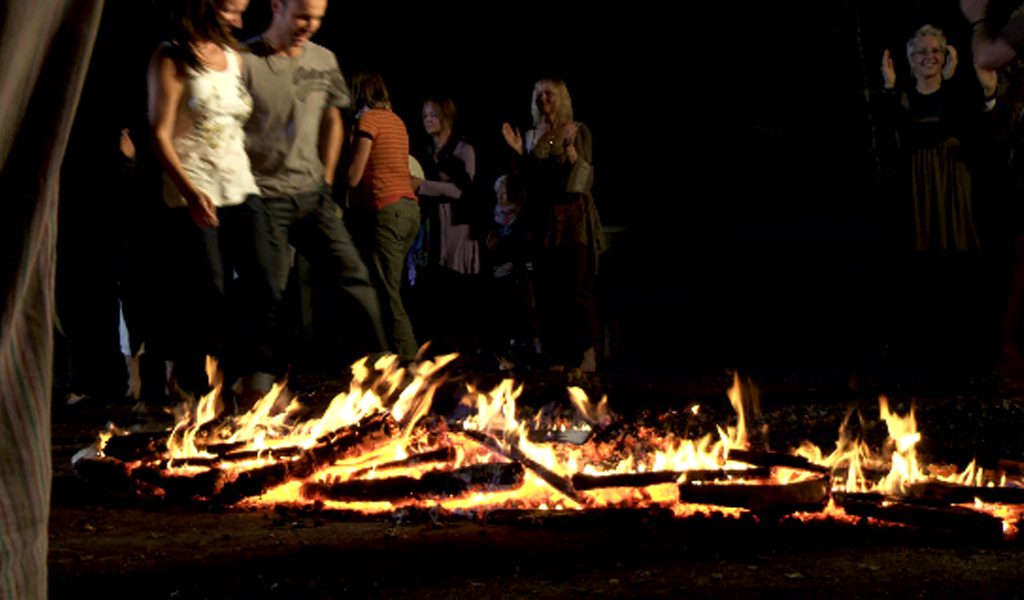The photograph captures a lively nighttime scene of a large group of people gathered around a sprawling, low-to-the-ground bonfire. The atmosphere suggests a social gathering where everyone appears to be enjoying themselves, as indicated by their smiles and casual, warm-weather attire consisting of short sleeves and tank tops. The wide, expansive bonfire is composed of embers and logs spread out on the ground, giving it a big but relatively low appearance with no high flames. In the foreground, a young man and a young woman stand close together, their arms around each other as they gaze at the fire. Other individuals can be seen clapping and possibly singing, with some walking around in the background. Despite the dark night setting making specific details indistinct, the image conveys a sense of communal joy and togetherness.